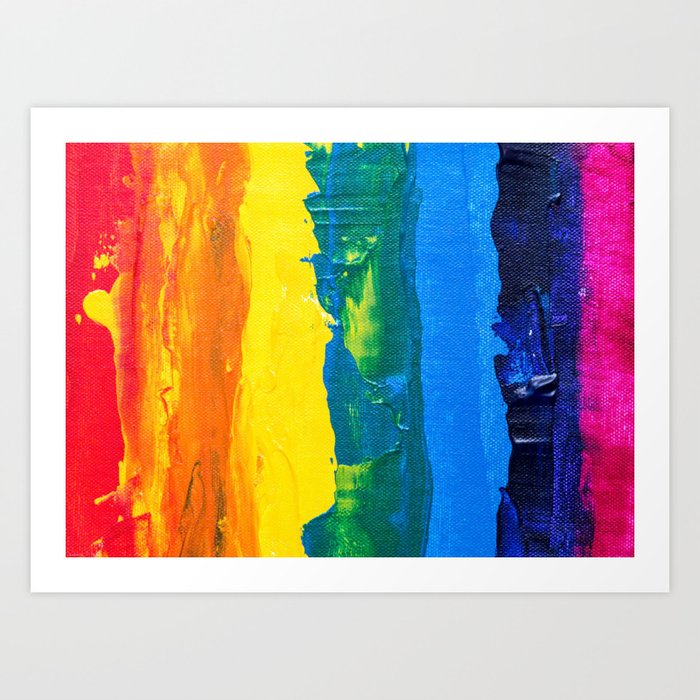This striking piece of abstract art is displayed on an off-gray wall, housed within a minimalist white frame. The horizontally oriented painting, laid against a white background, embodies a vibrant, abstract interpretation of a rainbow. It features a series of somewhat blended and overlapping vertical stripes: beginning with red on the left, merging into orange, then transitioning through yellow. This is followed by a mixture of yellow and blue creating green, evolving into a solid light blue, then a darker, indigo-like blue, and finally concluding with violet and touches of pink. The colors are distinctly vibrant yet seamlessly overlap at their edges, creating a harmonious blend that evokes the appearance of a spectral color gradient. Despite the messiness of the stripes' edges and the splotchy blending of colors, the overall effect is visually stimulating and beautifully eye-catching, making it a compelling centerpiece.